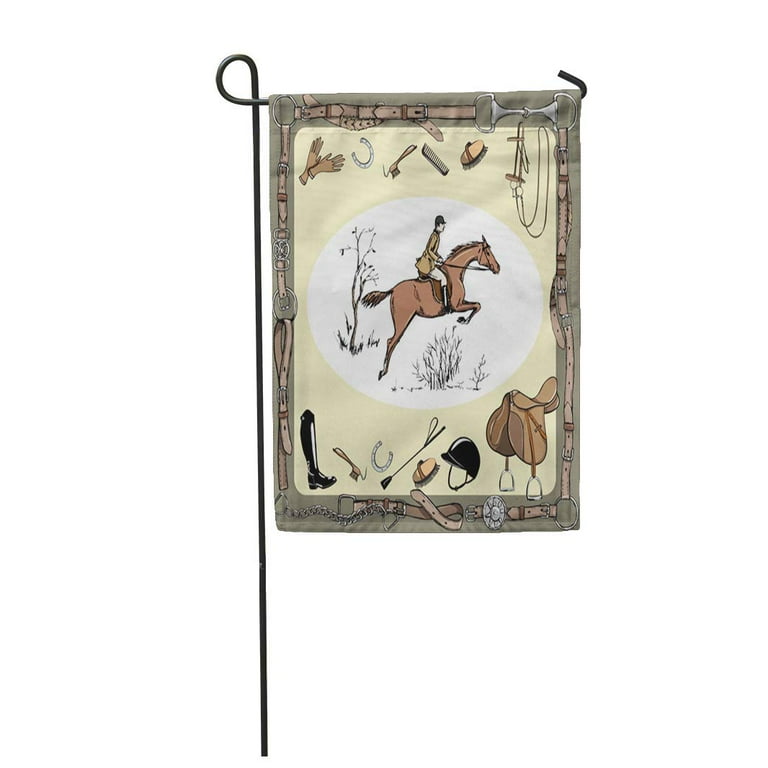This photograph features a garden or yard flag displayed on a decorative metal stake, set against a white background. The flag is bordered in light brown and showcases a central image of a dynamic brown horse, captured in mid-leap over a black bush. The horse's rider, dressed in a tan jacket and a darker riding helmet, is leaning forward and holding the reins. Surrounding this central scene, the flag is adorned with various equestrian-related items. Above the horse, there are illustrations of tan gloves, a horseshoe, and multiple horse brushes. Below, it features a black riding boot, a riding crop, a black helmet, and a tan saddle. The overall color scheme incorporates shades of brown, yellow, off-white, and black, with a hint of pea soup green, giving the artwork a straightforward and simple aesthetic.